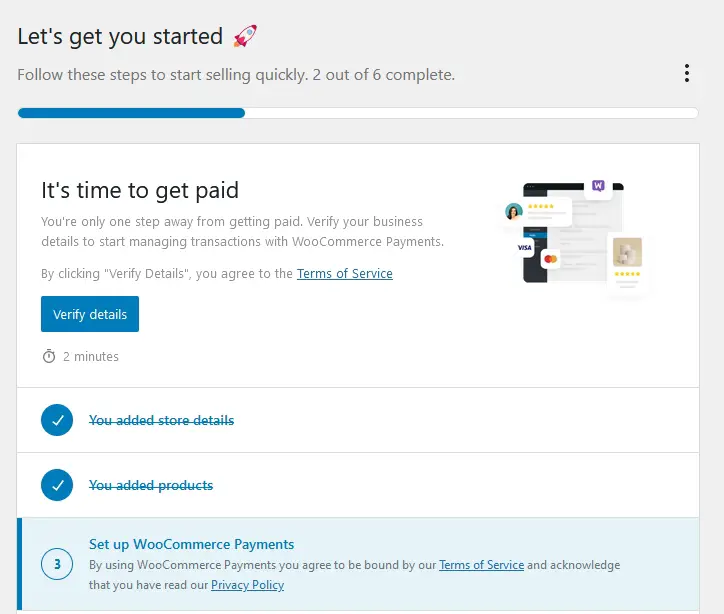The screenshot from the website presents a structured onboarding interface with distinct color sections and clear instructions. 

The top 2-inch section of the page is light gray, while a quarter-inch light gray border runs along the left and right sides. The content within this frame features a white background. At the top left corner, large black text prominently states, "Let's get started." Immediately below this, a graphic of a rocket ship, with red tips on both ends and a gray body, ascends towards the upper right.

On the left side of the page, the heading "Follow these steps to start selling" is displayed. Beneath it, a blue bar indicates progress with the text "2 out of 6 complete." Adjacent to the blue bar, on the right side, two black dots are aligned vertically.

Directly beneath this section, a header reads "It's time to get paid" in bold black text. Two less prominent black lines follow this header, providing additional context. Below this, a statement reads, "By clicking verify details you agree to the" with "terms of services" in green and underlined text, which links to more information. 

Towards the bottom left, a blue button labeled "Verify Details" is displayed. Accompanying this button to its left is a small stopwatch icon with the text "2 minutes" in black. A horizontal gray line spans the width of the section just below.

Further down, a blue circle with a white check mark and the text "You added store details" in blue, though struck through by a blue line, indicates a completed step. Another gray line divides this section from the next, where a similar blue circle with a white check mark signifies the step "You added products," also marked as completed with a strikethrough.

The bottom inch and a half of the page transitions to a light blue background with a dark blue border running down the right side. Centrally positioned on the left is a light blue circle containing a dark blue number "3," with adjacent dark blue text stating, "Set up WooCommerce payments." Below this heading, two lines of smaller black text provide additional details.

Overall, the interface is cleanly segmented, guiding the user through the step-by-step process with clear visual and textual cues.